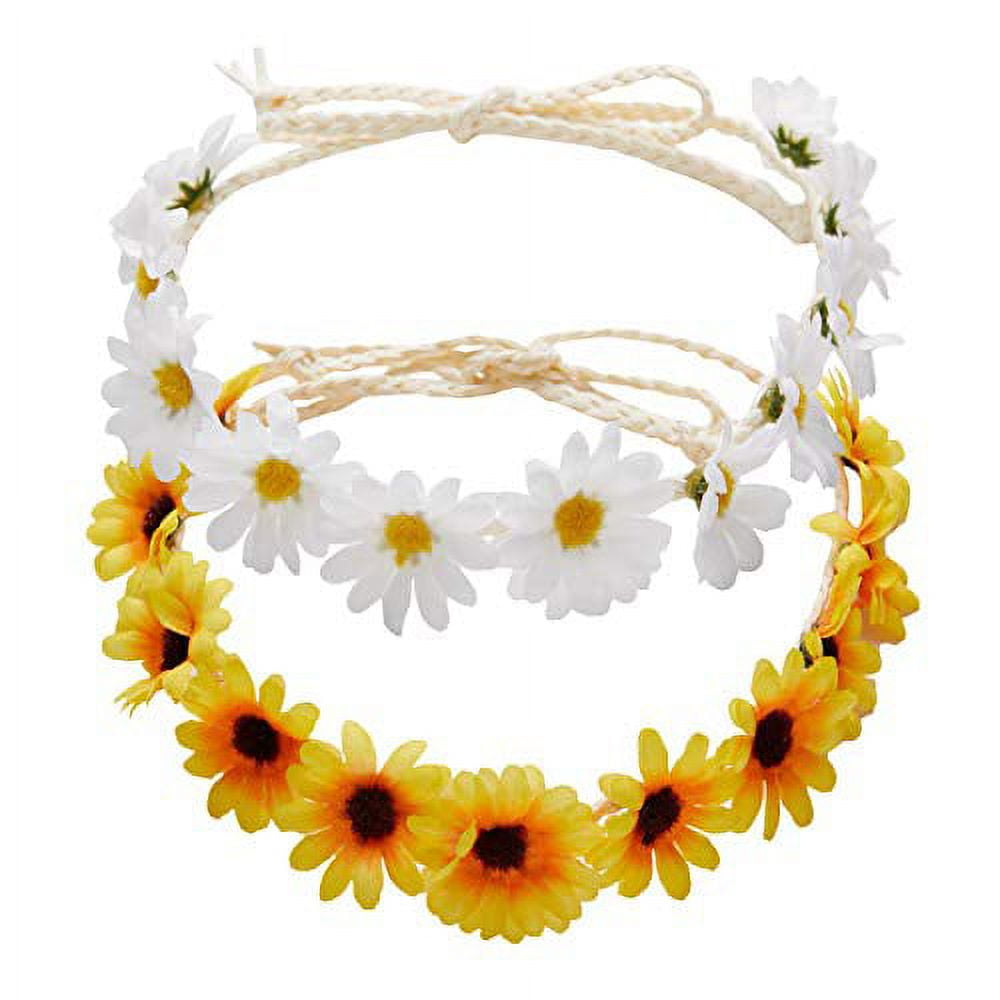This image features two floral headdresses made of thin beige braided rope, designed either as headbands or chokers, ideal for festival wear or social media advertisements. Both headdresses are depicted on a white background, arranged in an overlapping manner. The top headdress showcases 11 white flowers with yellow centers, covering approximately 75% of its front, leaving the back quarter bare with visible knotted twine. The bottom headdress resembles small sunflowers, featuring petals that transition from vibrant yellow at the tips to orange near the dark brown or black centers, creating a striking contrast between the two pieces. Both headdresses can be worn individually or together for a complementary look.